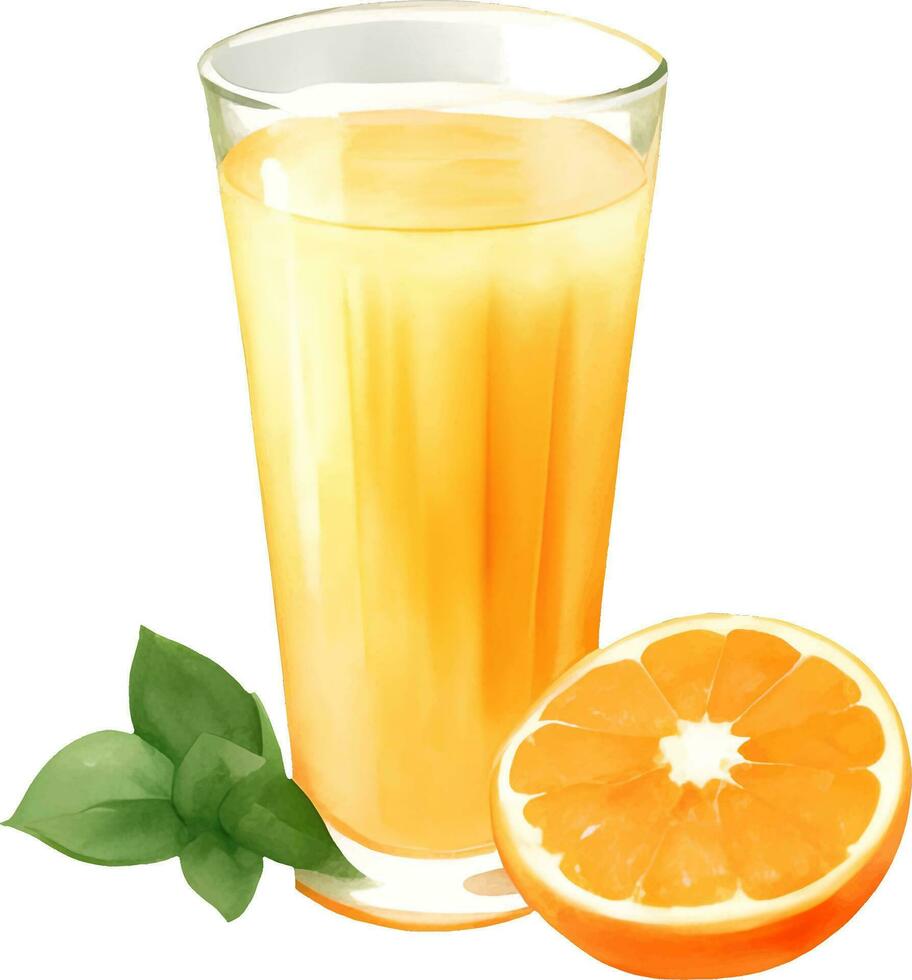This detailed and realistic illustration showcases a large, cylindrical glass of orange juice with a tapered base, wider at the top and narrowing towards a thicker glass base. The glass is filled almost to the brim with bright, vibrant orange juice, giving it an inviting and refreshing appearance. To the left of the glass, there are five green leaves, possibly mint, adding a fresh touch to the composition. On the right side of the glass, a juicy, ripe orange cut in half is strategically placed with the cut side facing up, further enhancing the vivid and luscious depiction. The overall style of the illustration is highly realistic, capturing every detail with striking clarity.